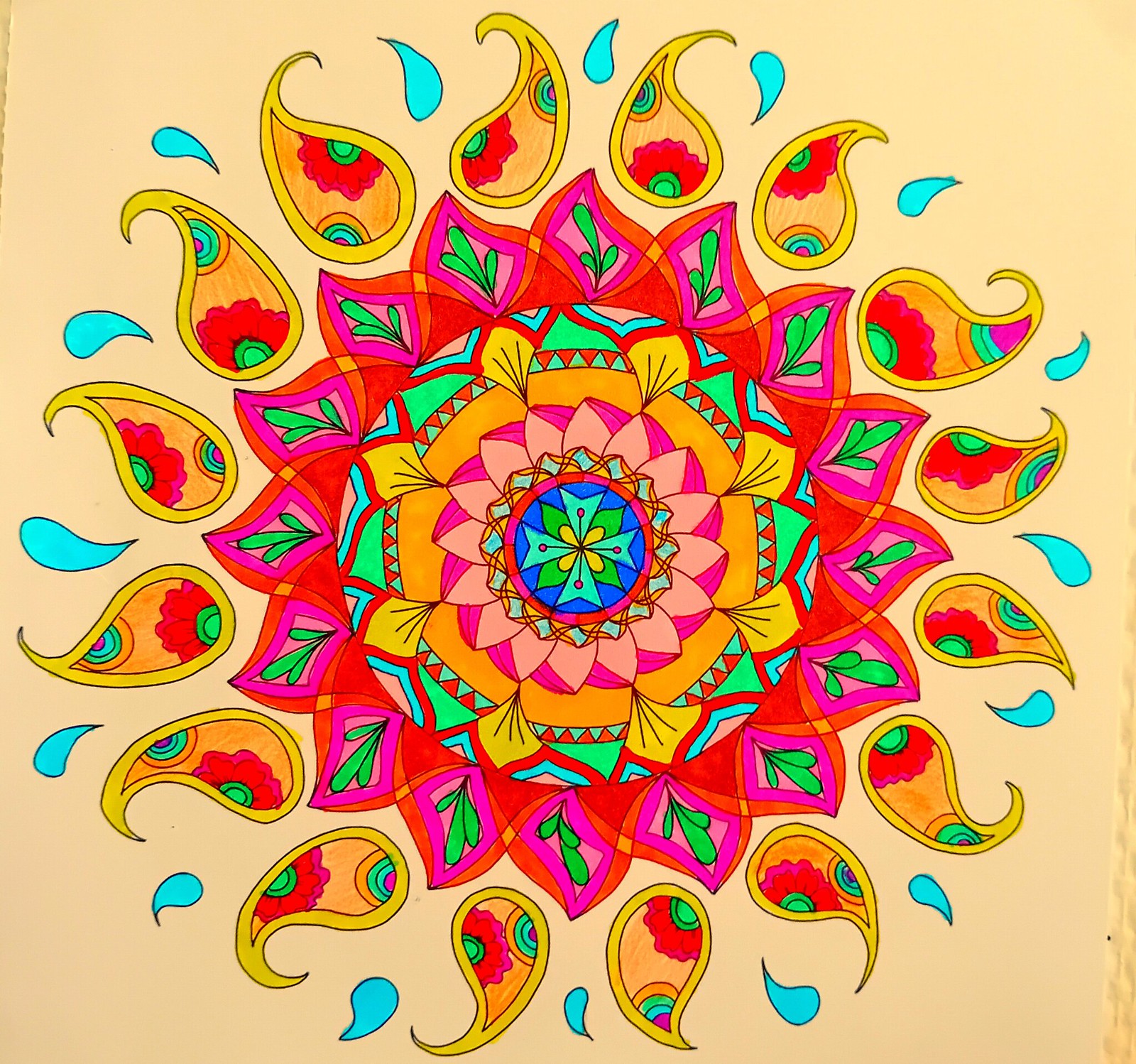This image depicts a highly intricate and colorful geometric pattern with a psychedelic feel, reminiscent of artwork from a coloring book or digital design. The central motif is a flower-like shape with jagged red outer edges and a green interior. At its core, there's a circular design featuring a teal cross set against a blue background, encircled by bands of light and dark pink, followed by orange, and then a lime green ring intertwined with red and blue lines. Yellow teardrop-shaped elements punctuate this vibrant center, adding to the complexity.

Surrounding the flower are numerous paisley teardrops with light teal raindrops adorning the outer edges. The overall pattern sits on a light beige background and incorporates a wide spectrum of colors, including pink, blue, yellow, green, purple, and orange. The detailing is rendered with thick pen and colored markers, enhancing its vivid, almost hallucinogenic appearance. This elaborate design fills the entire image area, creating an engaging visual that captures the eye with its multifaceted shapes and riot of colors.